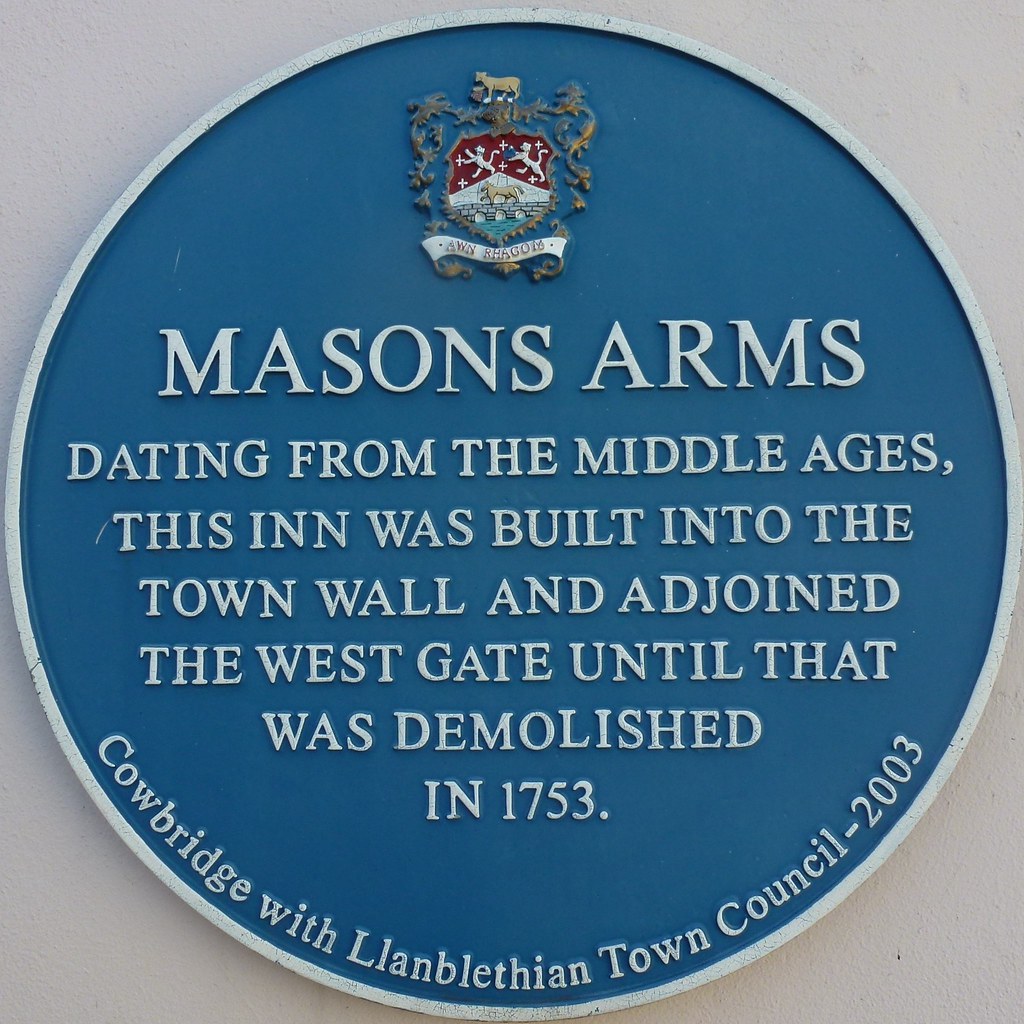This image shows a historical plaque installed on the side of a building. The plaque is circular with a silver outline and a blue center. At the top, it features a city crest designed as a shield with a banner underneath, displaying text in Latin. The crest includes two lions standing on their hind legs with their front paws extended, surrounded by crosses on a golden background, and a horse trotting across a bridge beneath the banner.

In the middle of the plaque, written in silver text, it says "Mason's Arms." A detailed description underneath states: "Dating from the Middle Ages, this inn was built into the town wall and adjoined the West Gate until that was demolished in 1753." At the bottom of the circle, curved along its edge, it reads "Cowbridge with Llanblethian Town Council, 2003."